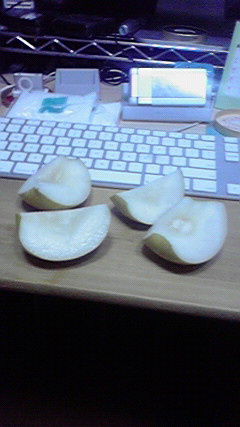The image captures a detailed scene of a workstation, likely in someone's home or office. In the foreground, resting on the light brown wooden desk, are four large, juicy slices of a cored green apple. Directly behind the apple slices stands a grayish keyboard, with flat, white keys. Further back on the desk, there's an assortment of Apple products including an older, silver iPod Shuffle and possibly a small portable speaker. Above the keyboard, a small monitor, which resembles a phone turned on its side, is visible. In the blurred background, additional items such as a silver wire rack and perhaps an iPod charger or stand can be partially seen. Dark colors dominate the ambiance, indicating the photo was taken indoors, possibly with a cellphone camera.